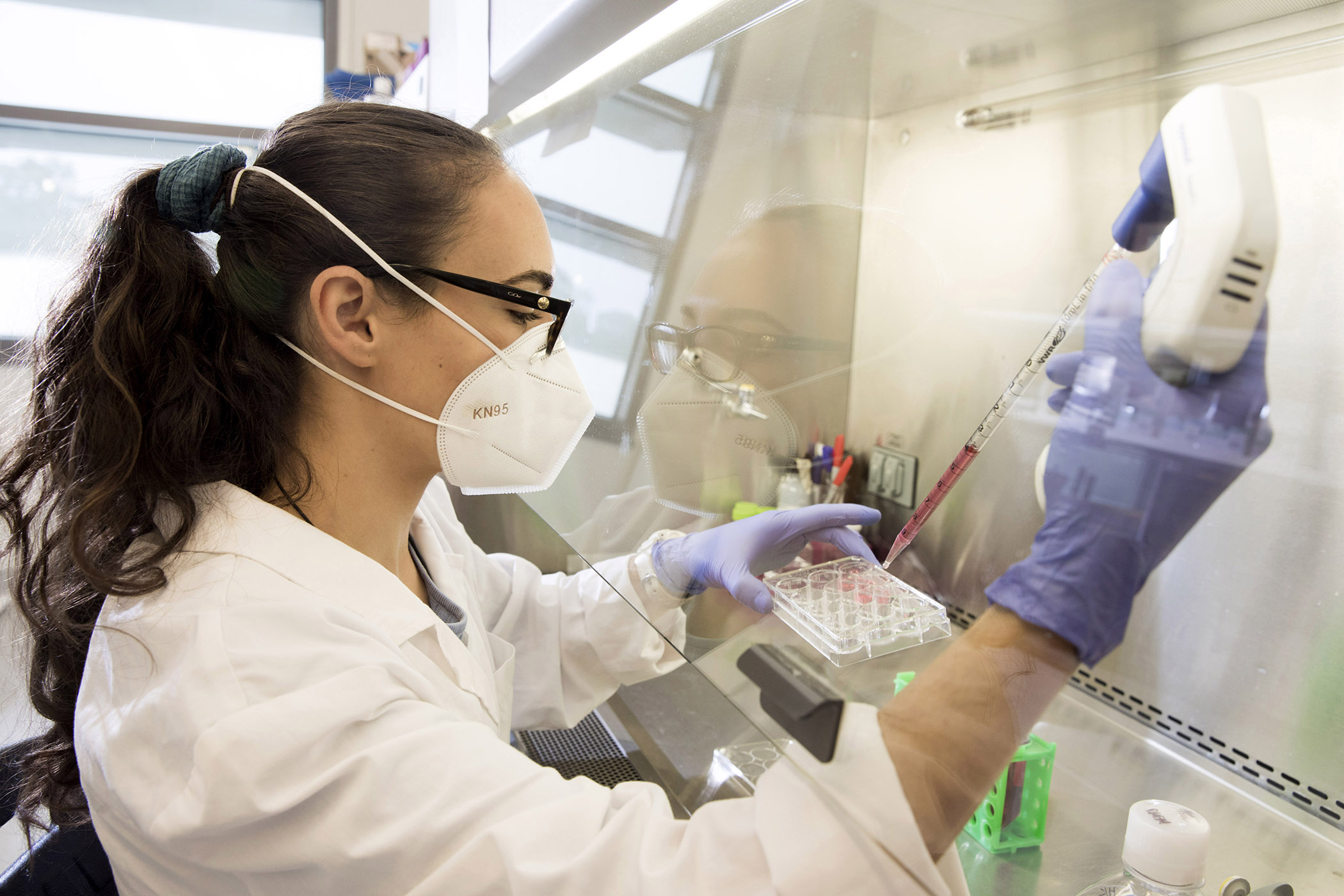The image depicts a woman, presumably a medical researcher or lab technician, in a laboratory setting. She is wearing a white lab coat, black eyeglasses, blue latex gloves, and a white KN95 mask. Her long, curly black hair is tied back in a ponytail with a scrunchie. She is seated and facing to the right of the photograph, working under a transparent protective shield. With her right hand, she holds an unusually large syringe or pipette containing a purplish-pink liquid, which she is meticulously injecting into a series of tiny vials encased in a tray she holds with her left hand. The scene includes various items on the shelves around her, such as a cup of pens and other indistinct medical equipment, reinforcing the laboratory environment. Her reflection can be seen in the protective plastic shield in front of her.